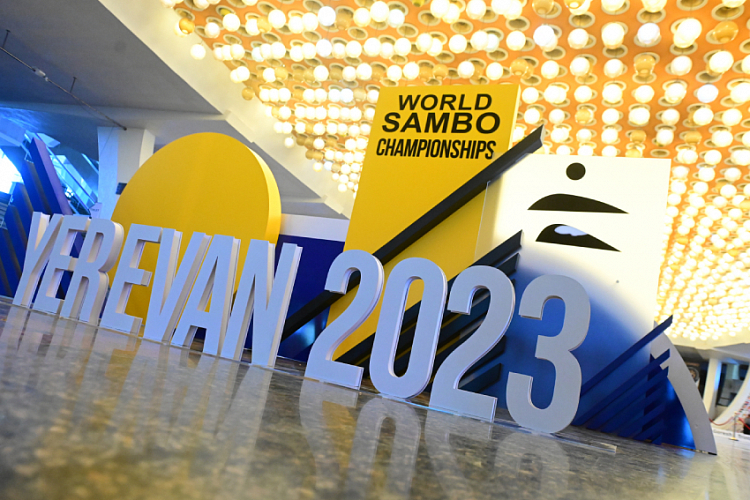This color photograph captures an entrance area of a convention center, showcasing a prominent and detailed 3D sign. The image is taken from the ground looking up, providing an angled perspective that highlights the glossy floor. The central focus is a large, multi-part sign with white block letters spelling "YEREVAN 2023" against a vibrant yellow background. Beneath this, another section of the sign reads "World Sambo Championships" in black text on a yellow rectangle. This entire display appears to mark the entryway, surrounded by the convention center's spacious atrium. Above, the ceiling features numerous bulbous yellow and white lights, enhancing the dramatic effect of the space. On the left side of the image, a white wall is visible, along with columns and escalators leading up to the second floor, further emphasizing the grand scale of the location. The combination of architectural details and the elaborate sign creates an inviting yet dynamic atmosphere for visitors.